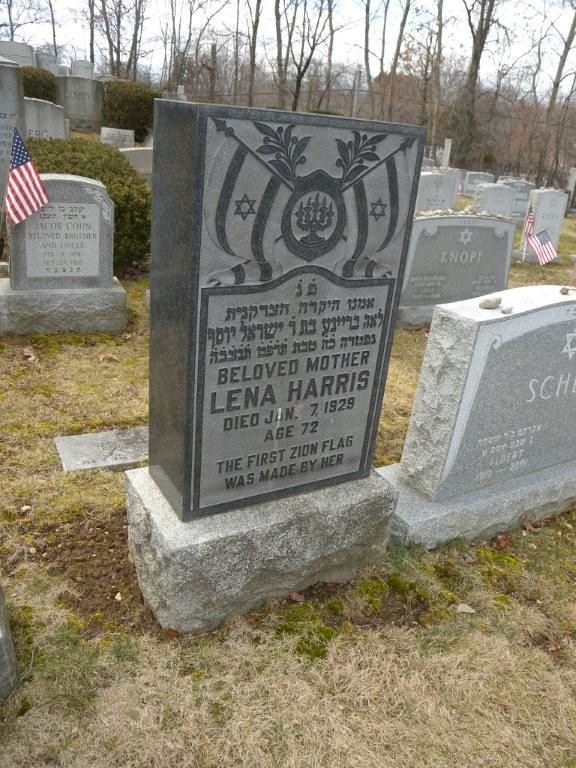This photograph features a prominent gray headstone, set upright on a marble slab, within a tranquil cemetery landscape. The headstone, primarily light gray with dark gray lettering, commemorates Lena Harris, who is described as a 'Beloved Mother'. The inscription details her death on January 7, 1929, at the age of 72, and notes the significant detail that she made the first Zion flag. The upper section of the headstone includes Jewish lettering and symbols: a menorah, two Zion flags adorned with Stars of David, and decorative elements in varying shades of gray. The cemetery backdrop reveals numerous other headstones dotting the scene, with a serene line of trees visible in the distance.